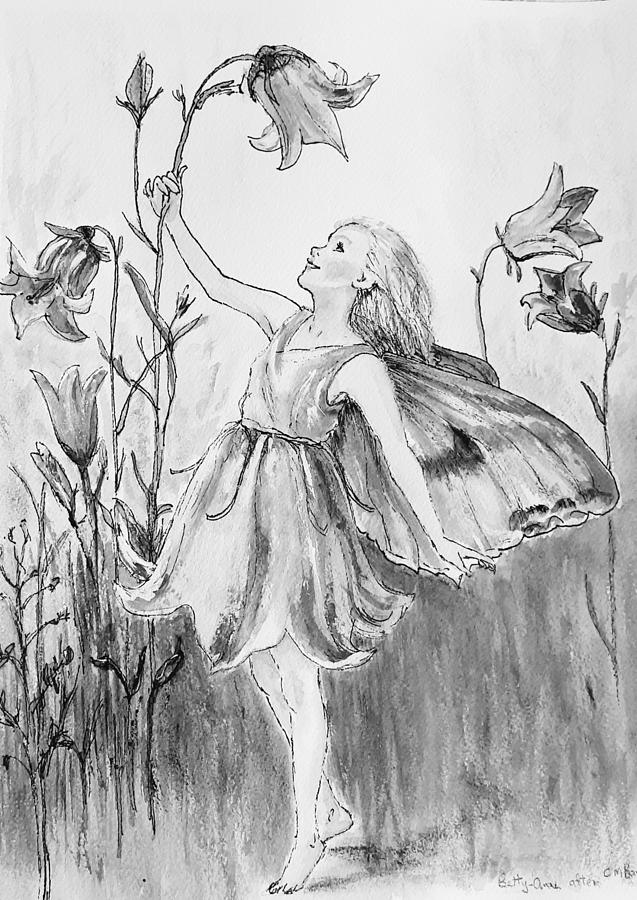The image is a detailed black-and-white sketch, likely created with charcoal or pencil, that captures a serene and enchanting scene from a fantasy or fairy tale setting. At the center of the illustration is a young girl who appears to be a fairy, indicated by her delicate butterfly-like wings emerging from her back. She is dressed in a knee-length, sleeveless frock that closely resembles flower petals, tied around the waist. The young fairy is barefoot and smiling as she gazes up at a tall, weaning flower that towers over her. She stands on her toes, one hand gently grasping the flower's stem while the other rests near her wings. Her long hair cascades down her back, adding to the ethereal atmosphere. Surrounding her are numerous tall flowers and blades of grass, emphasizing her tiny stature in this expansive, outdoor field. The sketch features meticulous shading, with the lower part of the image darker than the upper, enhancing the depth and texture. Overall, this charming illustration looks like it belongs in a fairy tale book, capturing a moment of whimsical, natural beauty.